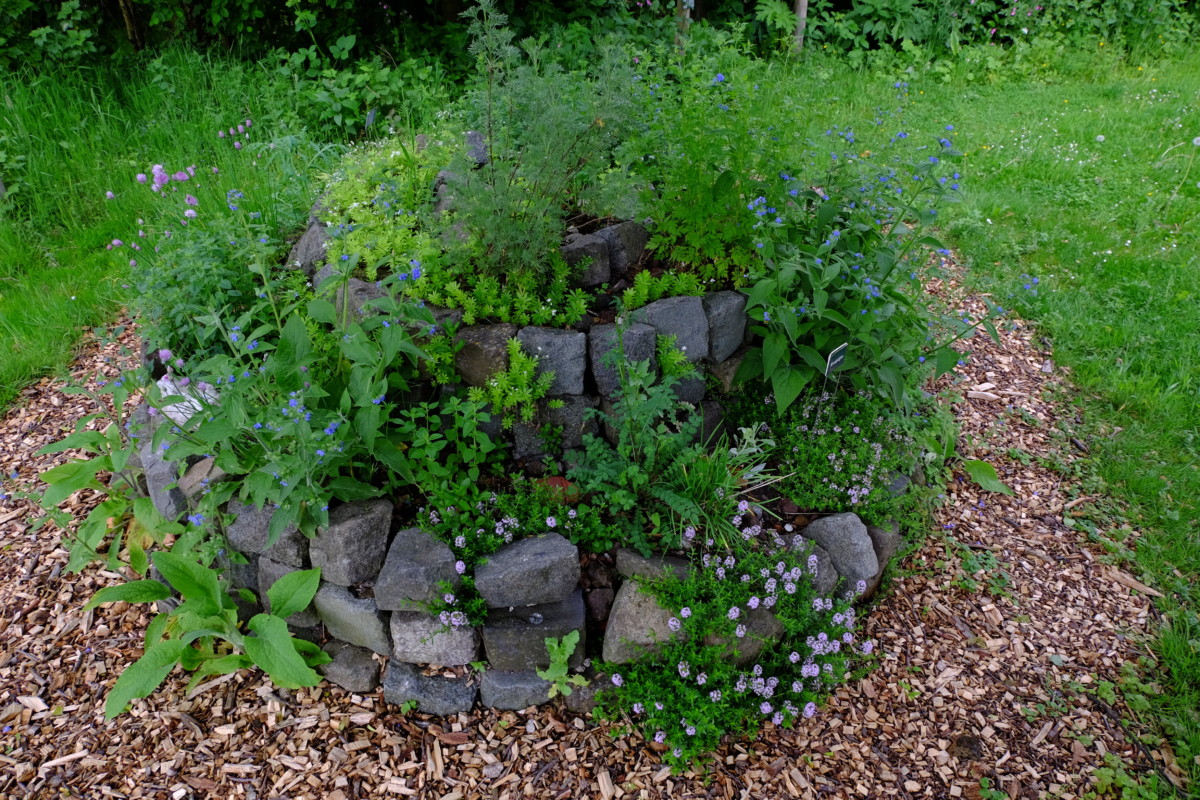The photograph showcases a meticulously arranged garden space, characterized by a concentric stone structure at its heart. This structure consists of several rings of stones, each stacked higher than the one below, forming a tiered design. Nestled within these stone rings are various herbs and flowering plants, including mint and colorful blooms of blue and purple hues, creating a lush herb garden. Surrounding the stones, a bed of light brown wood chips forms a circular pattern, adding a neat aesthetic touch. The outer boundary of this landscaped area transitions into a grass lawn, interspersed with some low-growing plants and weeds, highlighting the well-maintained yet natural charm of the garden.